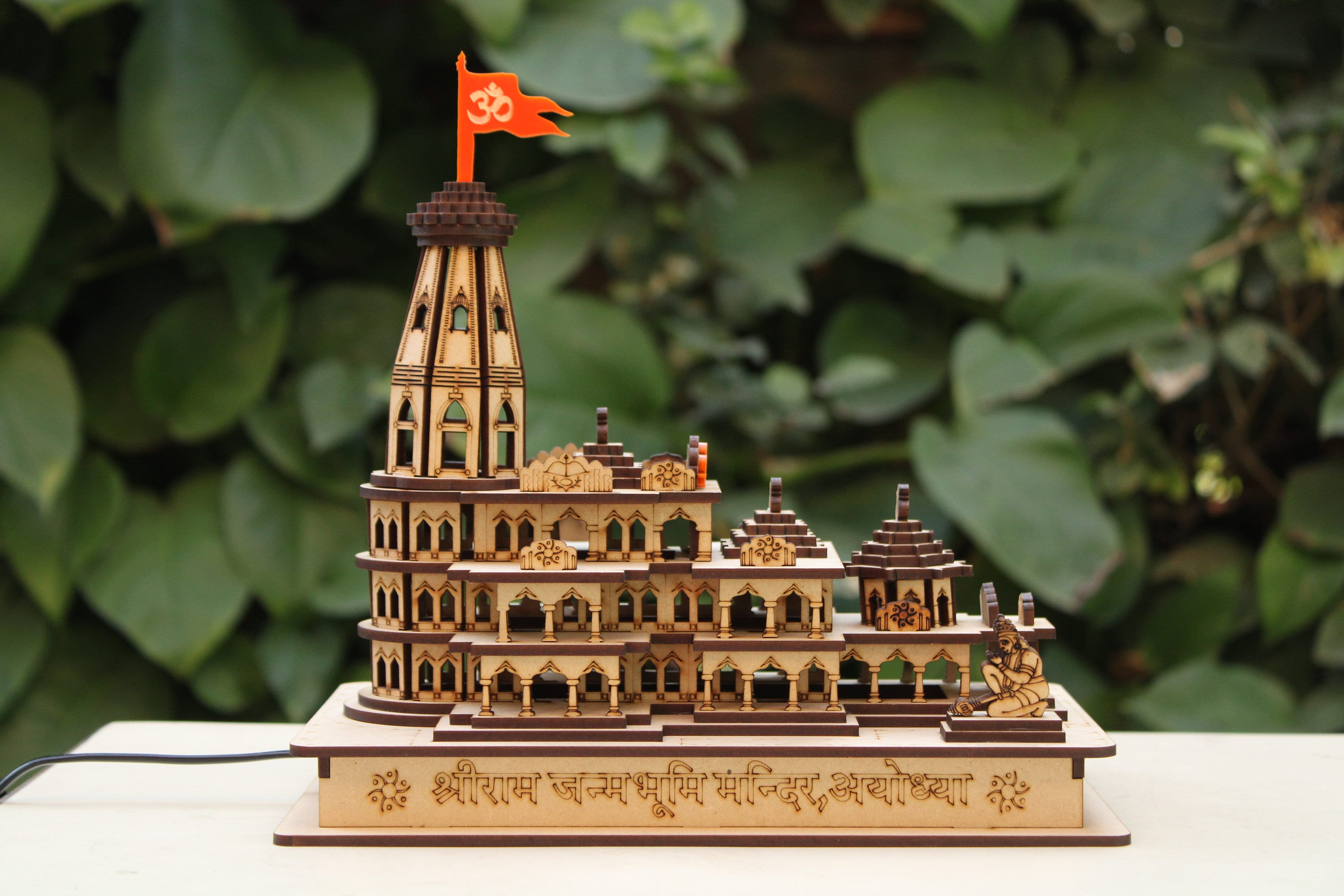This intricate scale model appears to depict a traditional Thai castle or temple, distinguished by the use of Thai script indicating its cultural origin. The entire structure is predominantly tan and brown, decorated with extensive architectural details. The castle features multiple levels, each adorned with ornate decorations and structures.

At the very top of the castle stands a prominent red flag, inscribed with Thai writing. Beneath the flag, atop the highest tower, a decorative arrangement of brown circular levels incrementally increases in size, creating a visually captivating pinnacle. The facade of the castle is marked by numerous windows and an array of columns on both the first and second floors, adding to its grandeur.

The second roof level and the third roof level each boast brown pyramid-shaped structures, each crowned with spire-like adornments, enhancing the temple’s classical Thai aesthetic. Additionally, situated on the second level is a small round building supported by a pavilion with columns, suggesting a place of contemplation or worship.

In front of the temple, a figure of a kneeling Buddhist deity further emphasizes the model's religious significance. Etchings and markings on the temple are distinctly spiritual, with one design resembling a sun accompanied by moon-like elements between its rays and a central circle. Another notable emblem on the third floor features the depiction of a bow and arrow with ivy flourishes beneath it.

In addition to these intricate details, the model includes small floral elements, notably a red flower visible from the front. An electric cord suggests that the model likely has an integrated lighting system to highlight its features.

Overall, this detailed scale model serves as an elaborate representation of what seems to be a temple or castle intended for construction, capturing the essence of Thai architecture and religious artistry.